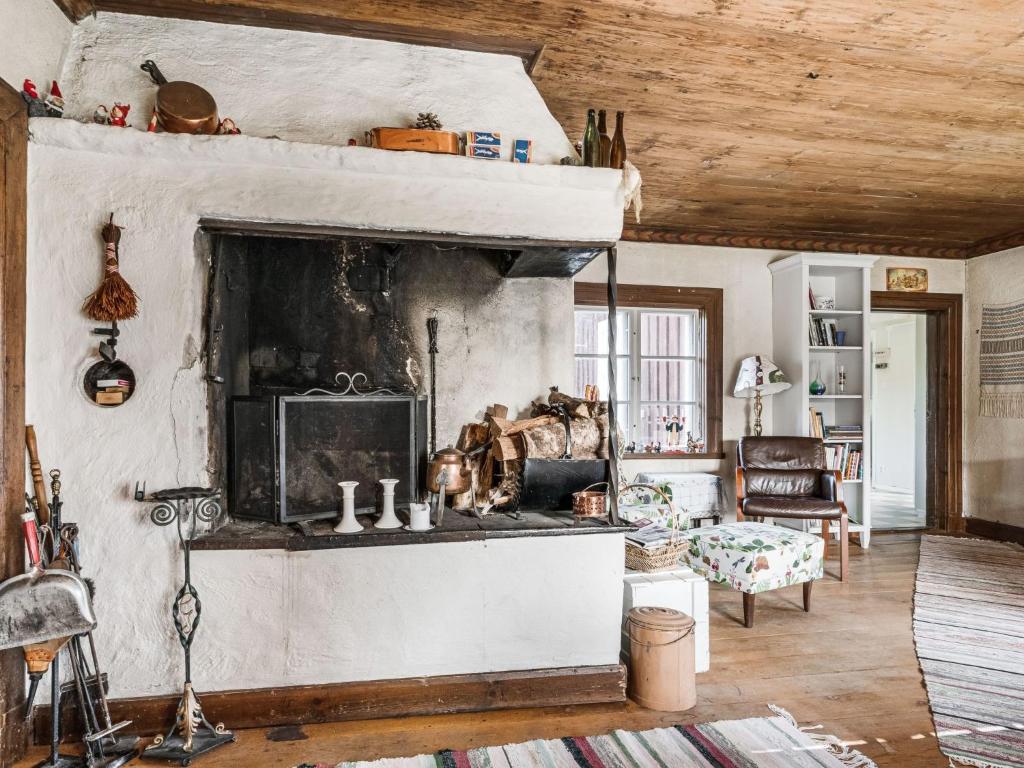This photograph depicts the interior of a rustic, homey room, showcasing a large, diagonally built fireplace situated in a corner cutout of the white, stucco walls. The imposing fireplace, which seems to feature a cast iron housing, extends into a large chimney that dominates the room. Directly in front of the fireplace is a pile of firewood, augmented by essential fireplace tools like a dustpan and fire poker. The room's ceiling and floor are crafted from matching wood planks, enhancing the rustic charm. The floor is partially covered by carpet runners that are adorned with white, black, and red stripes. Near the fireplace, a black leather reclining chair with an intricately floral-patterned ottoman invites relaxation. Adjacent to this cozy nook stands a white bookshelf and a lamp, completing the homely and inviting atmosphere of the space.